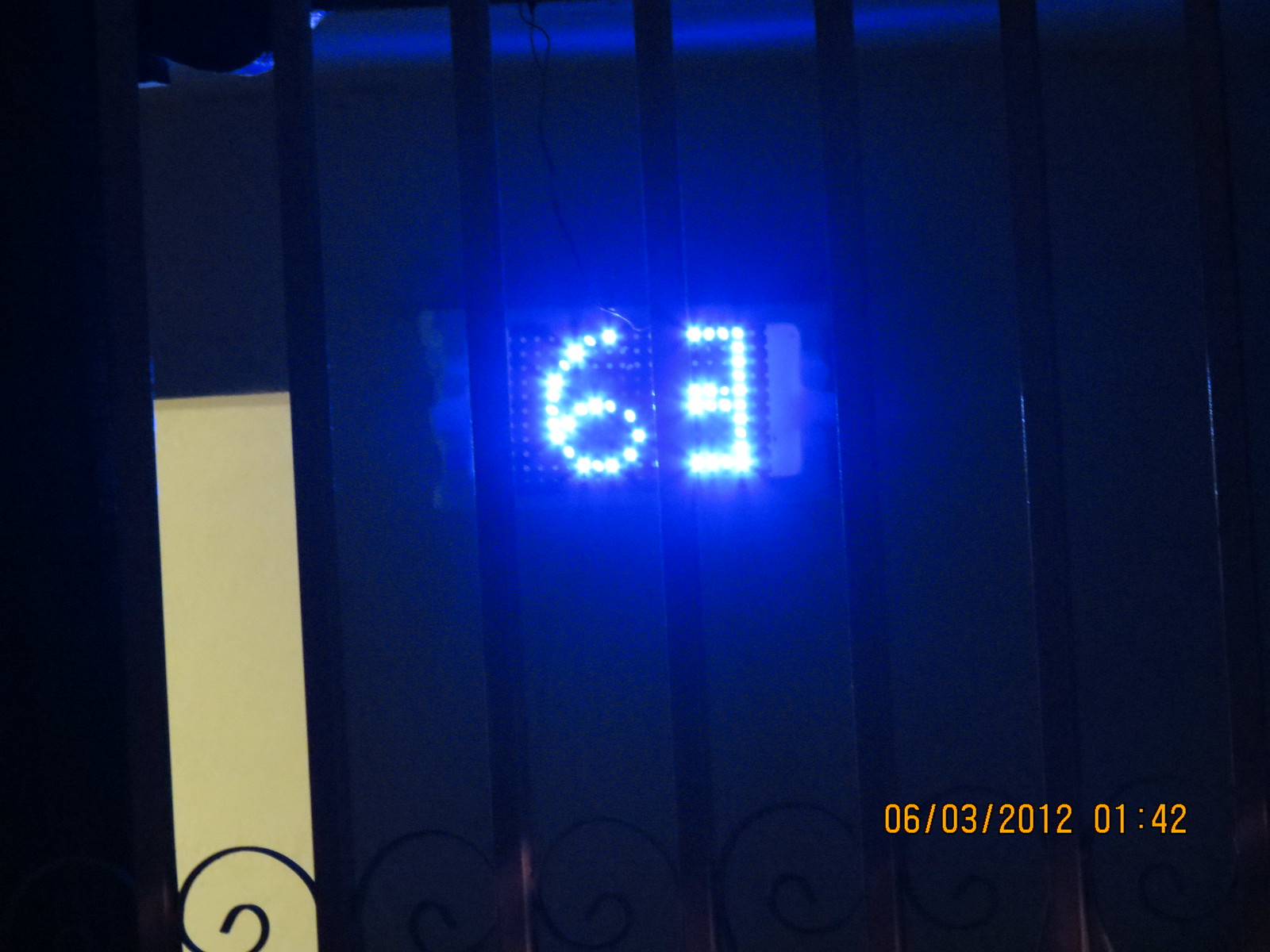This color photograph, taken at night, captures a section of a store window framed by iron security bars. On the left edge of the image, a bright white light illuminates part of the scene, casting a subtle glow on some decorative iron scrollwork at the very bottom. Behind the bars, a blue LED sign prominently displays the number "63," with the digit "3" featuring an unusual square shape, contrasting the rounded form of the "6." A time stamp at the bottom right corner of the photograph reads "06-03-2012 01:42," indicating the precise moment the photo was taken. The image is devoid of any other text or markings.